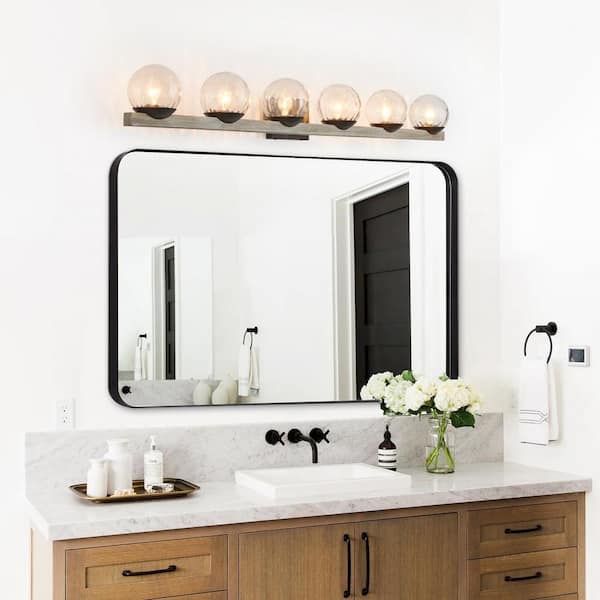This lifestyle image depicts a modern and elegantly staged bathroom, likely set up for an Airbnb listing or for a property sale. The walls are painted a pristine white, providing a clean backdrop for the chic decor. Centered in the square frame is a wide, black-framed mirror illuminated by an embankment of six globe lights that cast a warm yellowish glow.

Beneath the mirror, a sophisticated black faucet is mounted over a sleek, cream-white sink. The countertop is crafted from stunning grayish-white marble, extending slightly up to form a minimalistic backsplash. On the right side of the sink, a large vase with fresh white flowers adds a touch of natural elegance, while to the left, a tray holds three pump bottles, likely containing various soaps or lotions.

Adjacent to the sink on the wall, a round black towel rack holds a stylish white washcloth adorned with black designs, adding both functionality and flair. Below the countertop, brown wooden cabinets with black handles add a warm contrast to the otherwise monochromatic color scheme, providing additional storage space. The overall design is both functional and visually appealing, epitomizing contemporary bathroom aesthetics.